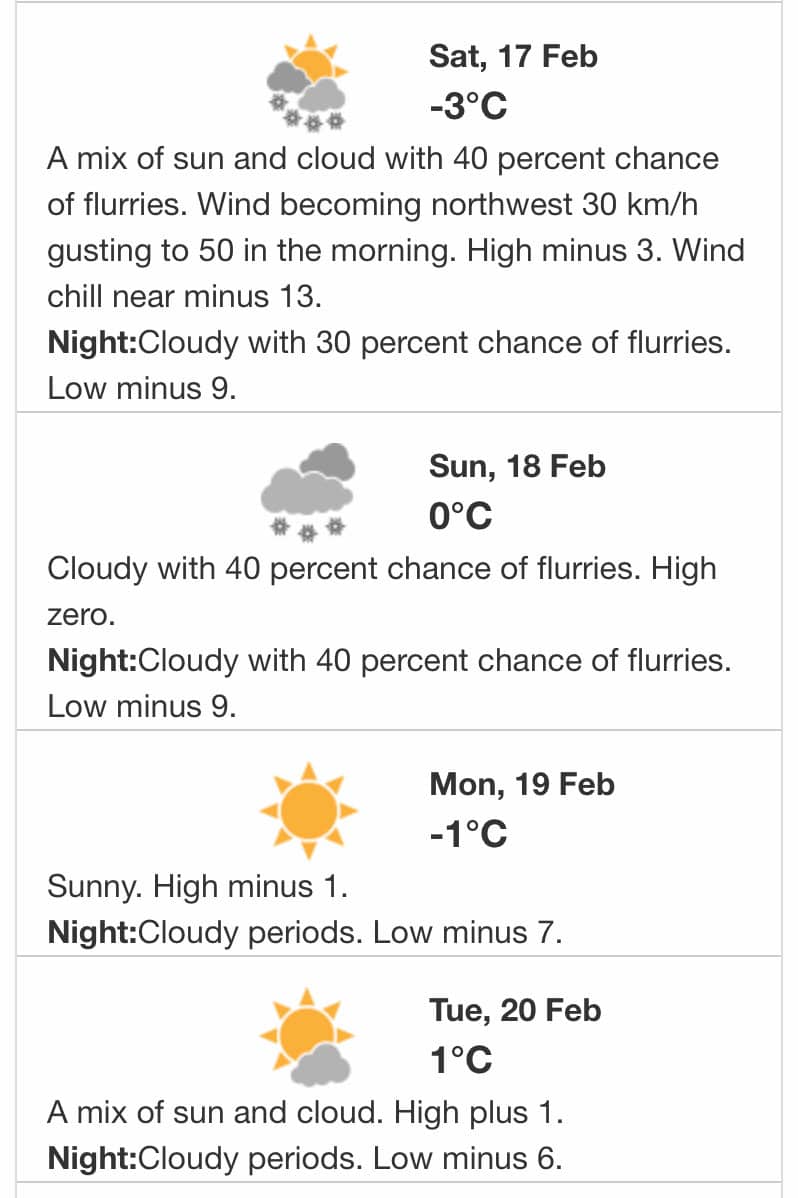The image presents a detailed weather report spanning four days, formatted in a rectangular layout divided into four sections, each representing a specific day.

**Saturday, 17 February:**
- **Day:** The top section indicates a high of -3 degrees Celsius. The weather is described as a mix of sun and cloud with a 40% chance of flurries. Wind will shift to the northwest at 30 kilometers per hour, gusting up to 50 kilometers per hour by the morning. The wind chill will feel like -13 degrees Celsius. 
- **Night:** The forecast predicts cloudy skies with a 30% chance of flurries and a low of -9 degrees Celsius.

**Sunday, 18 February:**
- **Day:** The second section shows a high of 0 degrees Celsius. There are images of clouds to the left of the date and temperature, indicating a weather prediction of cloudy skies with a 40% chance of flurries.

**Monday, 19 February:**
- This section also includes a weather report (details unspecified in the user's input, but implied to be similarly formatted).

**Tuesday, 20 February:**
- **Day:** The final section forecasts a high of 1 degree Celsius.

Each day's segment clearly distinguishes between day and night conditions, with comprehensive details on temperature, weather phenomena, and wind conditions, providing a thorough overview for the four-day period.